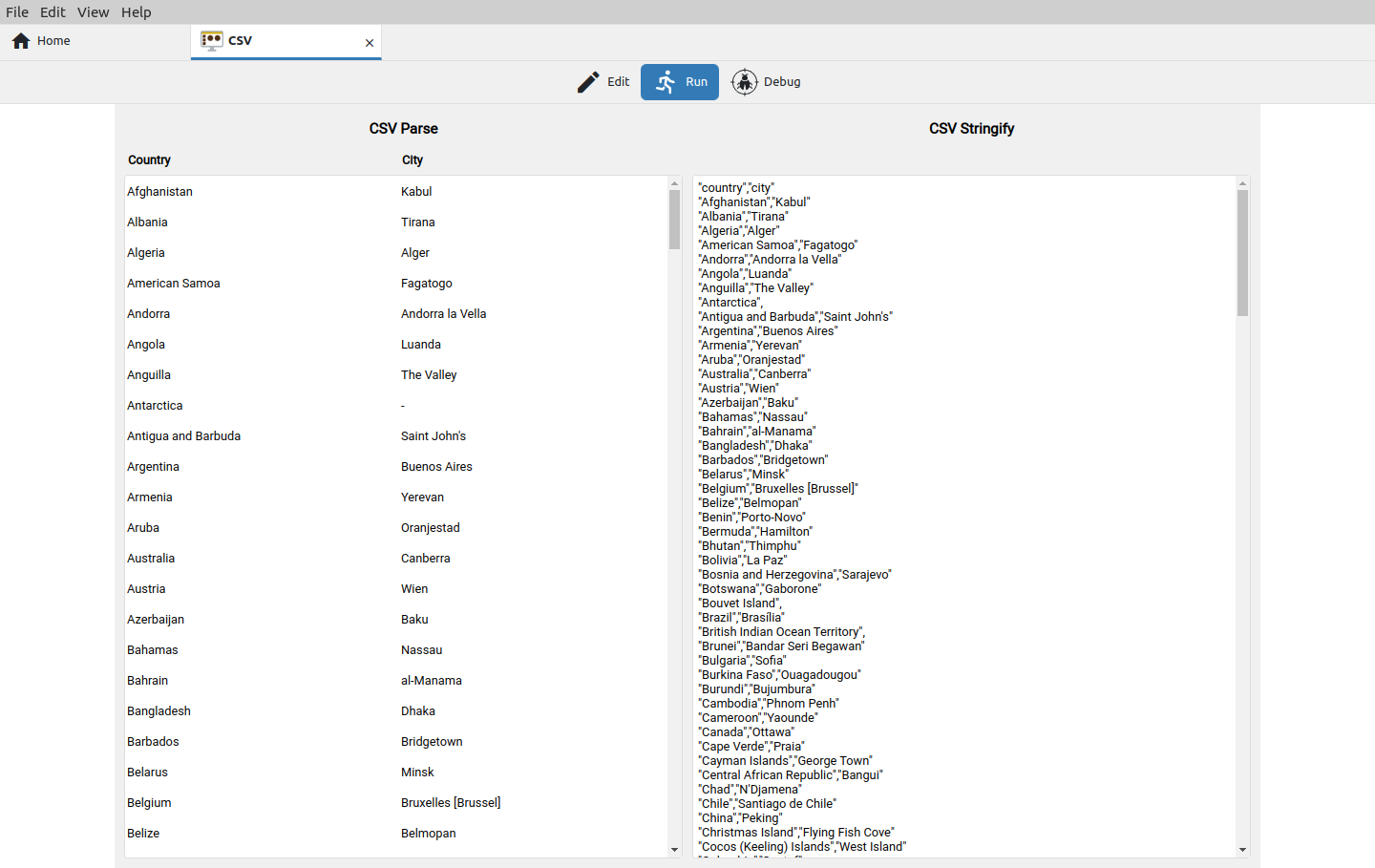The image depicts a screenshot of a website focused on parsing CSV data. At the top, there is a navigation menu with options including "File," "Edit," "View," and "Help," all situated within a gray bar. Just beneath this bar, the page is divided into several functional sections. 

On the left, there is a search bar that contains the text "CSV," with a "Home" label positioned above it. Below the search bar, a blue "Run" button is prominently displayed, accompanied by an icon of a person running. Adjacent to this button are various tool icons, including a crayon labeled "Edit" and a circular icon featuring a bug with the label "Debug."

In the central area, there is a dual-column layout showcasing parsed data under the heading "CSV Parse." The left column lists countries in alphabetical order, starting from Afghanistan and extending to Belize. Corresponding to each country, the right column displays related city names, also in alphabetical order. However, it seems that some data points may have been filtered out, as the column ends with entries starting with the letter "C."

The description indicates that after an operation—possibly a debugging process—the displayed data now accurately reflects the parsed countries and cities as expected.